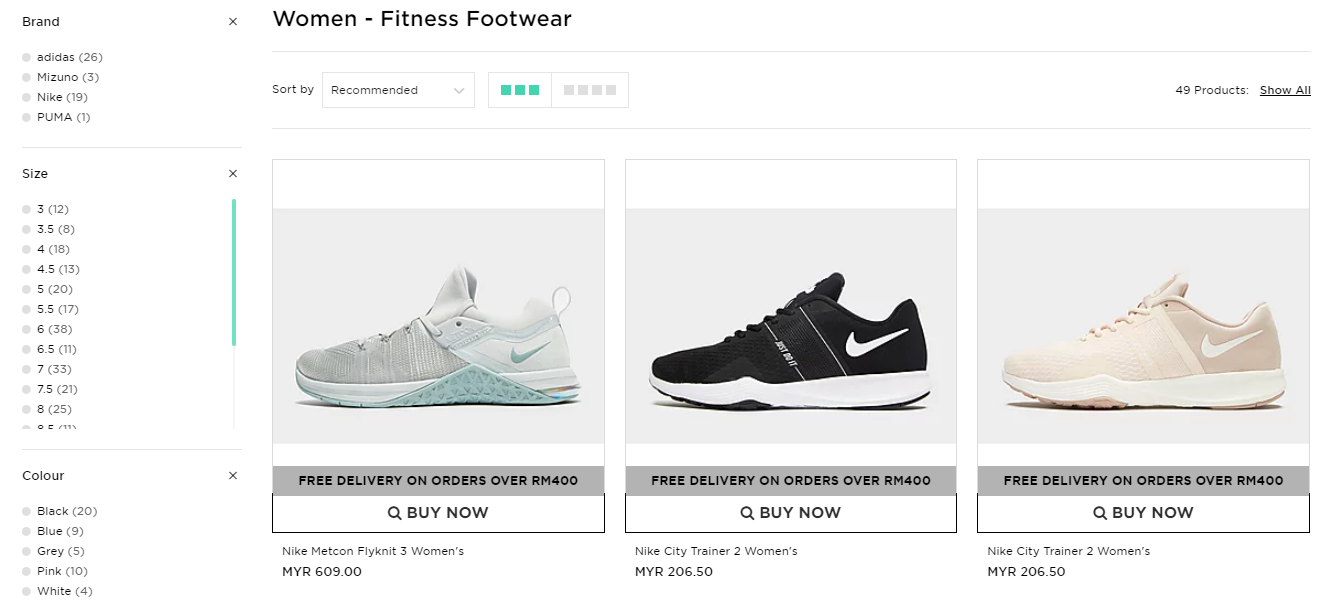Screenshot of a laptop viewing a women's fitness shoe shopping webpage in landscape mode. The white-background page prominently features three pairs of Nike sneakers against gray backdrops. At the very top, the header reads "Women-Fitness" in black text. Directly below, there is a filter option labeled "Sort by Recommendations," which reveals 49 products in total—currently displaying only three. These products can be expanded by clicking "Show All."

The first product is a pair of light-colored Nike sneakers with hints of blue and green. The middle product showcases a pair of black-and-white Nike sneakers. The third product is a taupe and peach-colored pair of Nike sneakers. Each product description includes "Free delivery on orders over RM400" directly above a "Buy Now" button.

Detailed product captions are as follows:
1. Light-colored sneakers: "Nike Metcon Flyknit 3 Women's, MYR609."
2. Black-and-white sneakers: "Nike City Trainer 2 Women's, MYR206.50."
3. Taupe and peach sneakers: "Nike City Trainer 2 Women's, MYR206.50."

On the left-hand side of the webpage, users can filter products by brand, size, and color options.